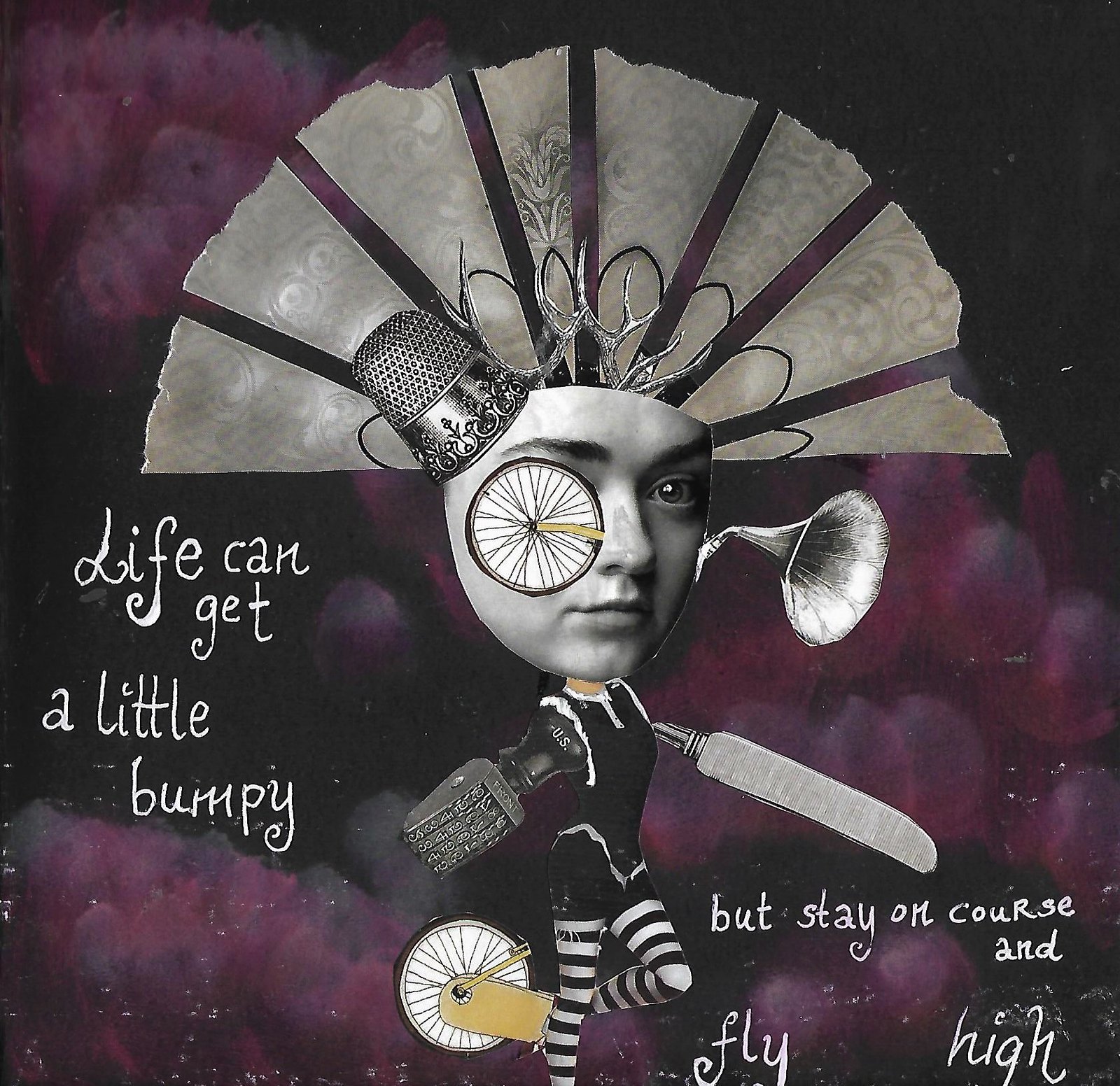The image is a striking piece of abstract collage art, combining black-and-white photography, illustration, graphic design, and typography. The format of the piece is square, with a dark purple, galaxy-like background featuring random cloud patterns. At the center of the composition is the face of a young woman facing to the right, seamlessly integrated with various surreal elements that give the artwork a gothic and eclectic aesthetic. 

Her right eye has been replaced with a line art bicycle wheel, while an old-fashioned gramophone horn emerges from the right side of her head. On the left side of her head, a silver thimble covers her ear, complemented by multiple fan shapes in light gray extending outward. Her right arm is depicted as a silver butter knife, and her left arm is an old-fashioned rotary stamper. The woman is adorned with black and white stockings or pants, and a bicycle wheel serves as her left foot, with the pedal visible.

Text in white script overlays the image, adding a poignant message. On the left side, the words "life can get a little bumpy" are written, while at the bottom right, the phrase continues with "but stay on course and fly high." This collage is a creative and modern work of art, blending fantastical elements with motivational typography.